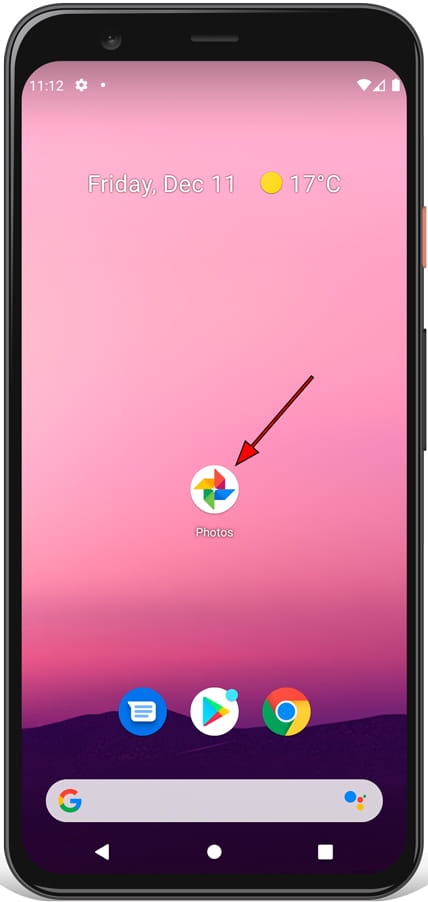The image showcases a realistically rendered photograph of a smartphone, highlighting the screen prominently. The phone's outer frame, appearing more digitally rendered than photographed, is dark grey and black, and features two buttons on its right side. A small pink button is positioned higher up, with a larger black button below it.

The smartphone screen is illuminated, displaying a serene background of a light pink and purple sky above a dark purple, smoothly rolling mountain range at the bottom. Centered on the screen is the Photos app icon, a white circle with a colorful pinwheel in front of it, comprising yellow, green, blue, and red colors. The icon is labeled "Photos," with a digitally added red arrow pointing diagonally downwards from the upper right corner towards the icon.

At the bottom of the screen are three additional icons arranged from left to right: a blue circle with a white messenger bubble, a white circle with the Google Play logo, and a circle displaying the Google Chrome logo. Below these icons lies a Google search bar. The top of the screen provides contextual information, indicating that it is Friday, December 11th, with a weather status of 17 degrees Celsius and sunny conditions.